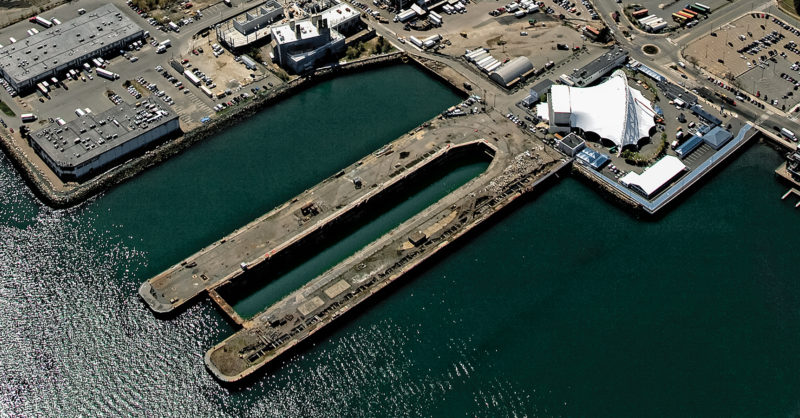This image captures an aerial view of an industrial port area, likely taken from a plane or helicopter. The scene is dominated by several industrial buildings with gray roofs and extensive parking lots filled with numerous cars and trucks. These structures and lots are situated adjacent to a green-blue body of water. Notably, two lengthy piers extend from the shore into the water, indicating a hub for shipping and docking activities. Towards the bottom right of the image, there is a large, distinctive white tent-like structure. The overall atmosphere is industrial, characterized by concrete surfaces and the bustling activity typical of a shipping port.